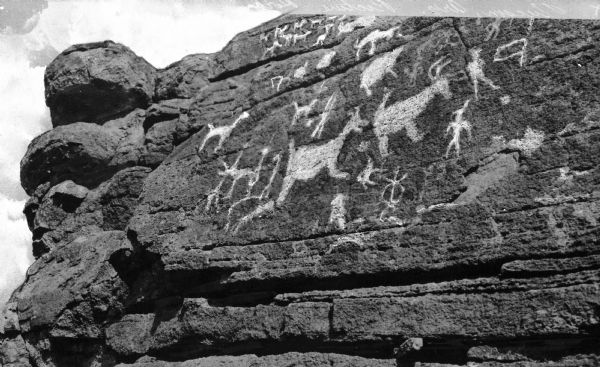This black-and-white photograph captures a large, rocky outcropping, likely situated in the American Southwest, adorned with ancient petroglyphs. Dominating the image, the dark rock extends from the bottom left to the top right, vertically striated with indented lines that give it a rugged texture. Centered on the rock face are detailed etchings of animals, possibly deer or ram-like creatures, characterized by discernible bodies, four legs, and varied ear positions, all appearing to move in a rightward succession. Below and to the right, stick-figure representations of people are visible, some seemingly engaged in a primitive ball sport. These ancient drawings, which include at least a half dozen animal figures and additional markings, evoke the artistic expressions of prehistoric peoples. The backdrop features a partly cloudy sky in the top left and faint outlines of distant mountains, enhancing the timeless and majestic feel of this striking archaeological scene.